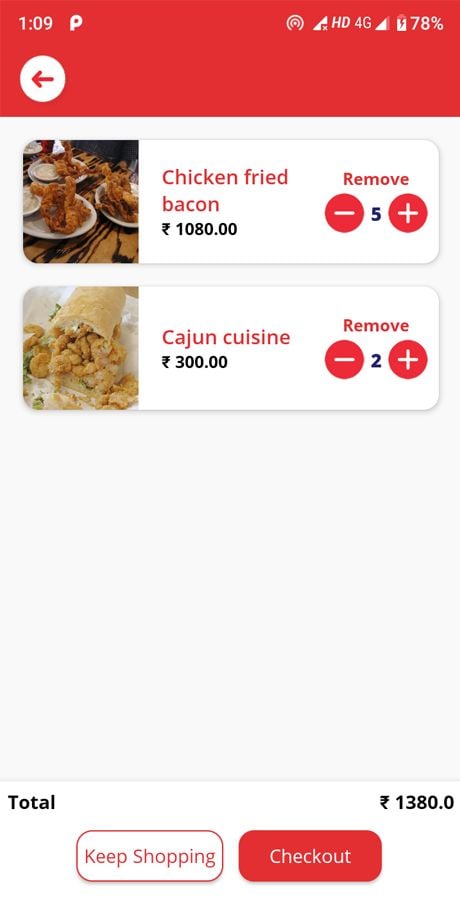**Detailed Description of the Screenshot from a Food Ordering App:**

The image is a screenshot of a mobile phone using a food ordering app, likely DoorDash or a similar service. The interface displays a foreign currency, which seems to be an East Asian currency, though the specific unit is not familiar. At the top of the screen, there is a red banner.

**Status Bar Details:**
- A white "P" icon for one of the notifications.
- Hotspot is activated.
- Connectivity is turned off.
- The phone displays "HD 4G" with nearly full signal strength (one bar shy of full).
- Battery level is at 78% and currently charging.
- The phone's information section indicates "109."

**Main Screen Details:**
Underneath the red banner, which includes a white circle with a red arrow on the left-hand side, is the primary interface of the ordering app displaying the user's cart.

**Cart Details:**
1. **Chicken Fried Bacon:**
   - Image: Small picture of chicken fried bacon on the left.
   - Price: 1,080 units of the currency.
   - Quantity: User has added 5 of this item.

2. **Cajun Cuisine - Shrimp Po'boy:**
   - Image: Small picture of a shrimp po' boy on the left.
   - Price: 300 units of the currency.
   - Quantity: User has added 2 of this item.

**Total and Options:**
- The total amount for the order is 1,380 units of the currency.
- Two buttons are available at the bottom:
  - A white button with "Keep Shopping" in red text.
  - A red button with "Checkout" in white text.

The clean organization and detailed display of items in the cart provide a clear overview of the user's order, making it easy to proceed with the final steps of the transaction.